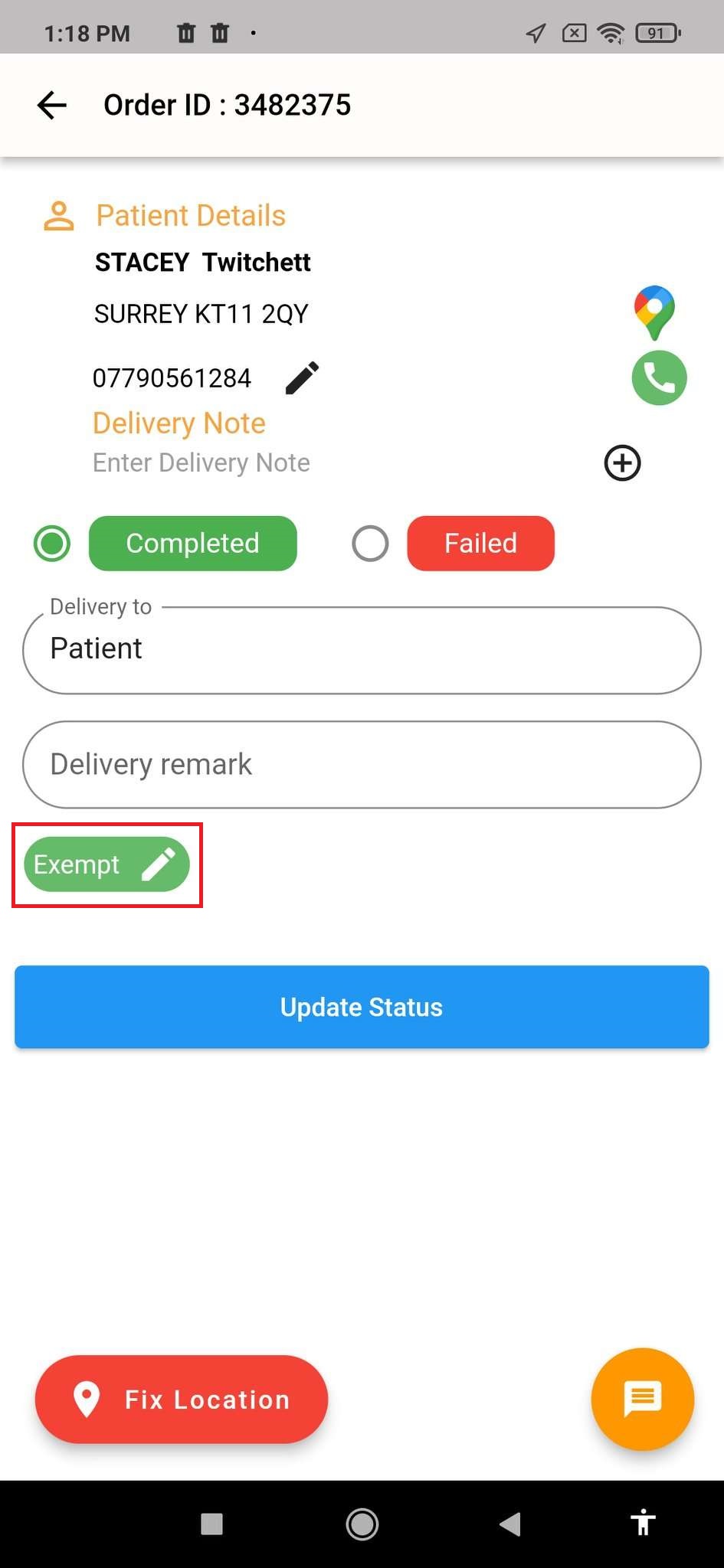The image on the phone screen shows various interface elements and details, giving an impression of a delivery app or service. 

In the top left corner, the time is displayed as 1:18 p.m within a shaded gray square. To the right of the time, there are multiple icons: two which appear to be trash icons, a location symbol, a square symbol with an X in the middle, a Wi-Fi signal icon, and a battery icon.

The main content area of the screen displays an order with the Order ID 3482375. This is presented on a white background with an arrow pointing to the left near the top. Below the Order ID, under a header labeled "Patient Details" in orange and accompanied by a person icon, is the name "Stacy Twitchett" along with the address "Surrey KT11 2QY" and the phone number "07790561284." Next to these details is a small pencil icon which suggests the option to edit.

Further down, there is another orange header labeled "Delivery Note," prompting to "Enter delivery note." Nearby, a location icon and a green circle with a white phone icon are visible, as well as a white circle outlined in black with a black plus symbol in the middle, indicating additional actions or options.

Towards the bottom of the screen, there's a section highlighting the delivery status, offering two options: "Completed" in green, and "Failed" in red. The "Completed" option is highlighted. Information below that includes "Delivery to: Patient" and "Delivery Remark," followed by a button or selection "Exempt" which is outlined in red with a pencil icon beside it. There's also a blue bar showing the option to "Update Status."

At the very bottom of the screen, there's an orange text labeled "Fixed Location" with an orange circle containing a white message note icon to the right of it. Additionally, several icons at the bottom of the screen include a square, a circle, an arrow pointing to the left, a person icon, and a black bar.

This detailed layout suggests a comprehensive interface likely used for managing and completing delivery tasks.